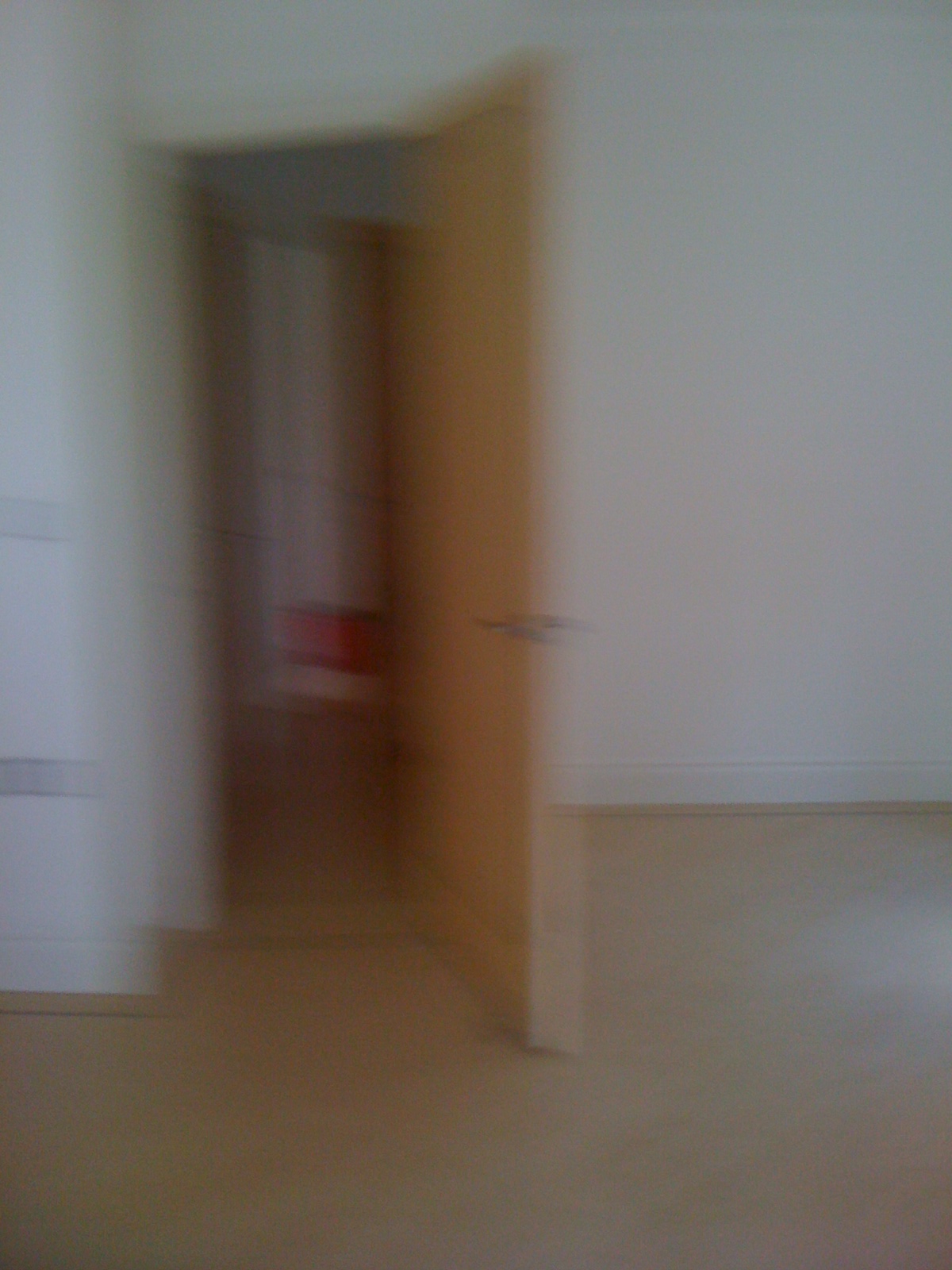This photograph, though blurry and out of focus, captures an indoor scene centering around a partially open, beige-colored door. The door, which appears slightly ajar, reveals a metallic handle protruding on both its interior and exterior sides. Through the doorway, a white-tiled wall becomes visible, accentuated by a distinctive red strip running along its lower portion. The left side of the door shows another wall aligned with it, before it abruptly turns left, creating a perpendicular angle. At the rear of the scene, a further wall can be glimpsed, painted white. The floor is of a tan-gray hue, providing a subtle contrast against the predominantly light-colored walls.